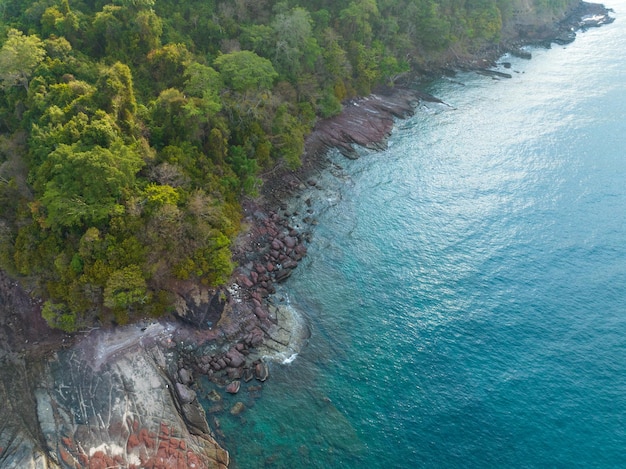This aerial photograph captures a striking scene of a very vibrant blue body of water, which could either be a lake or an ocean. The water dominates the upper right corner of the image, cascading down to the left and occupying roughly the bottom right half of the frame. The shoreline along this body of water is characterized by a mix of dark, black rocks and lighter, brown rocky sections. On the bottom left, there's a noticeable gray rocky area of the shoreline.

Behind this rugged shoreline, the terrain rises into a dense, lush forest. The greenery is composed mainly of various shades of green trees with some dead trees interspersed. The forest is thick with bushes and underbrush, creating an impenetrable, dense coverage that leaves little room for movement beneath the canopy. There are no tall pine trees visible; it's a complete, verdant expanse of forest that appears difficult to access.